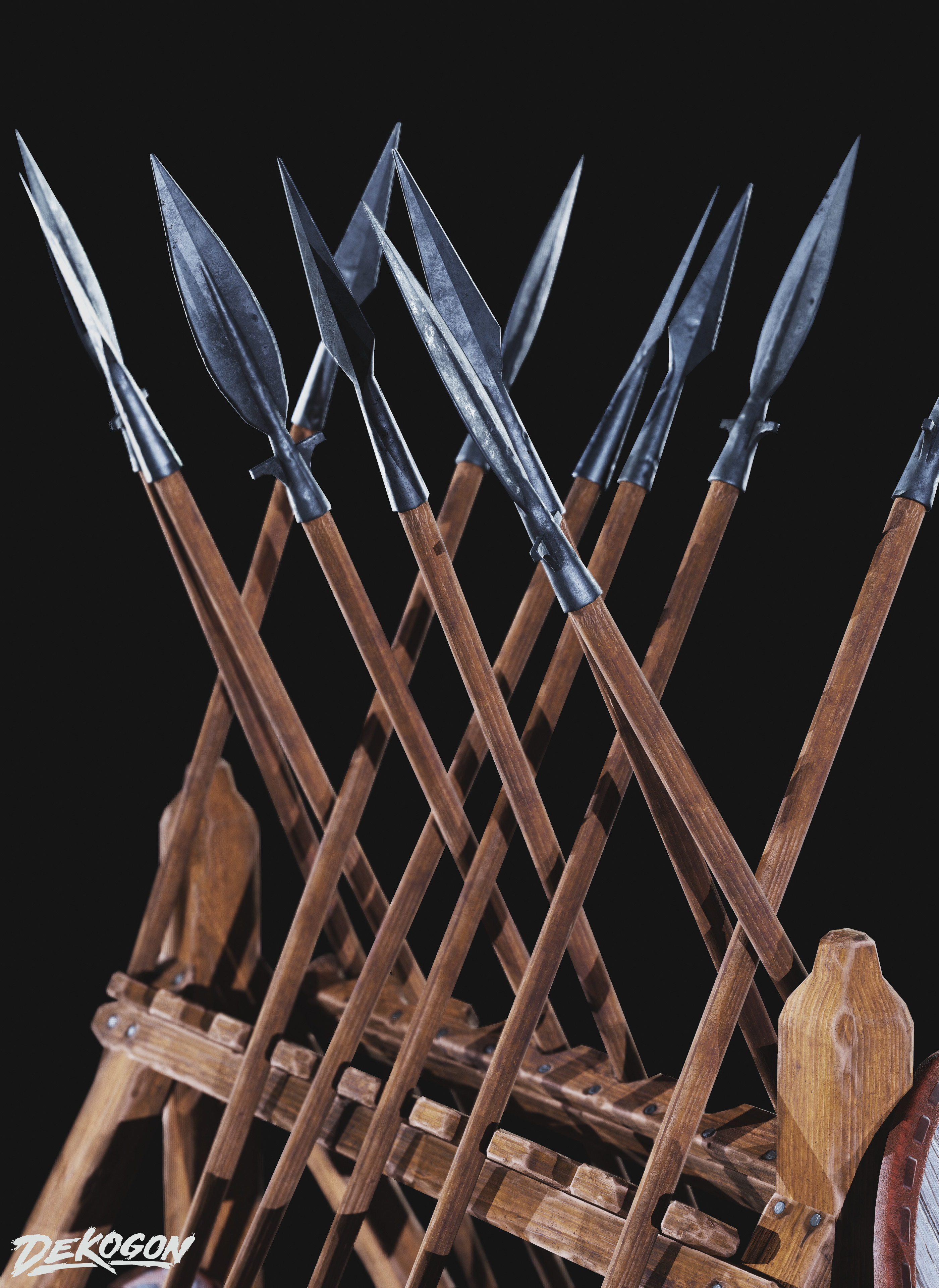This vertical color digital illustration presents a realistic depiction of a wooden spear rack, crafted with meticulous attention to detail. The rack features prominent grooves on either side of the top bar, which securely holds an array of spears. The spears are arranged with precision, positioned diagonally opposite one another, creating an intricate diamond pattern at the center of the image. Each spear has a sturdy wooden handle and a sharp, spade-shaped point reminiscent of the spade suit in a deck of cards. The overall palette is dominated by rich, dark tones, enhancing the dramatic effect of the scene. In the bottom left corner, the text "DEKOGON" is prominently displayed, signifying the brand or creator of this striking illustration, which appears to be a promotional artwork for these finely crafted spears.